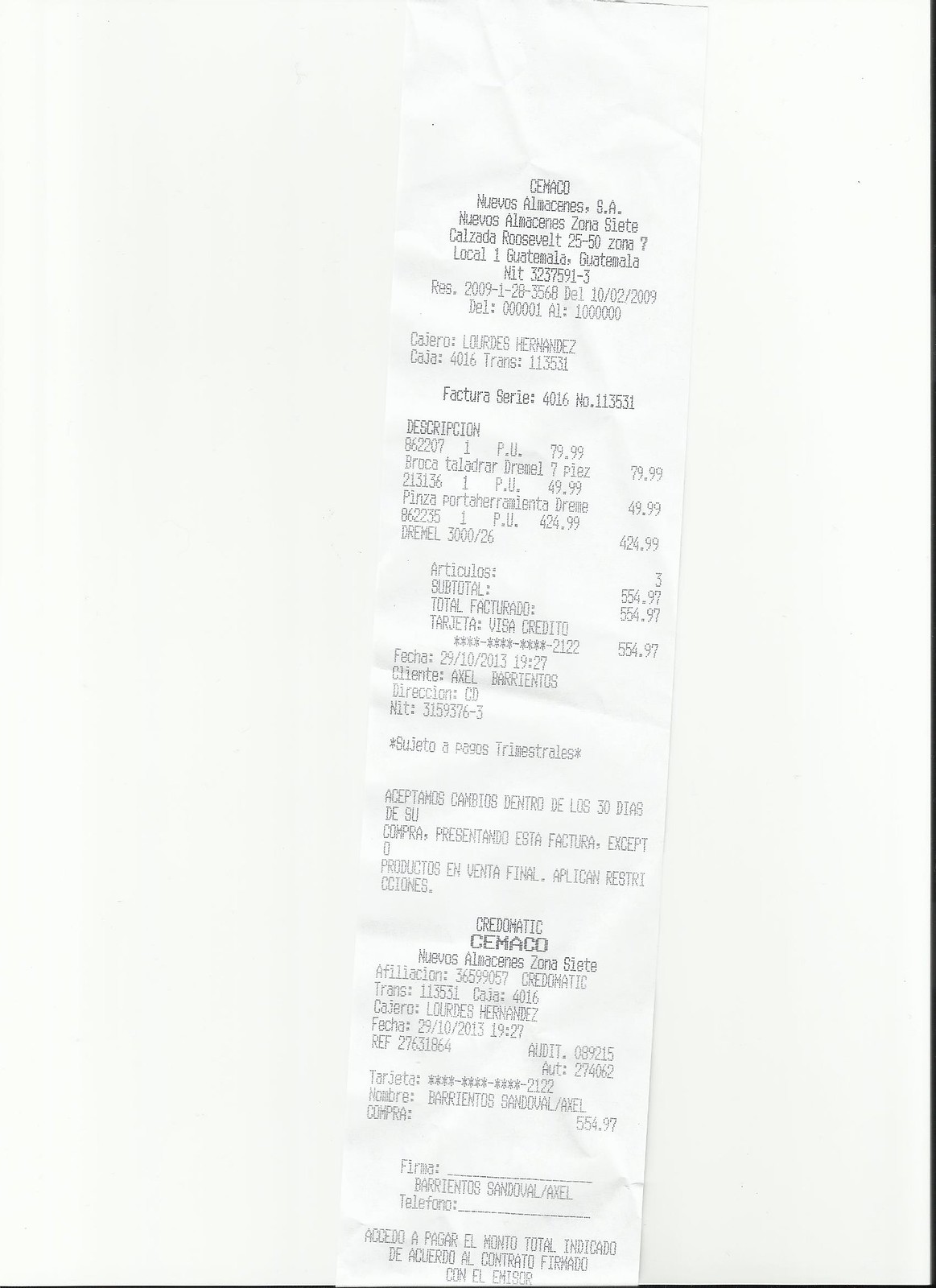The image is a detailed scan or photograph of a receipt from Camaco Nuevos Almacenes S.A., a store located in Guatemala City, Guatemala. The receipt documents a transaction for several items, including a Broca Taladrar Prey Tool 9 P.S. and a Pinza Port Jaramenta Dremel, among possibly other purchases, with individual prices listed as $79.99, $49.99, and a significant purchase of $424.99 totaling to $554.97. This amount was paid using a Visa credit card ending in 2122. The transaction was processed by a cashier named Lourdes Hernandez at register 4016, with the transaction number 113531. The date and time of purchase are clearly indicated as October 29, 2013, at 19:27 hours. The description includes meticulous details about every aspect of the receipt, down to the signed area at the bottom and the fact that the image was likely kept for documentation or tax purposes.